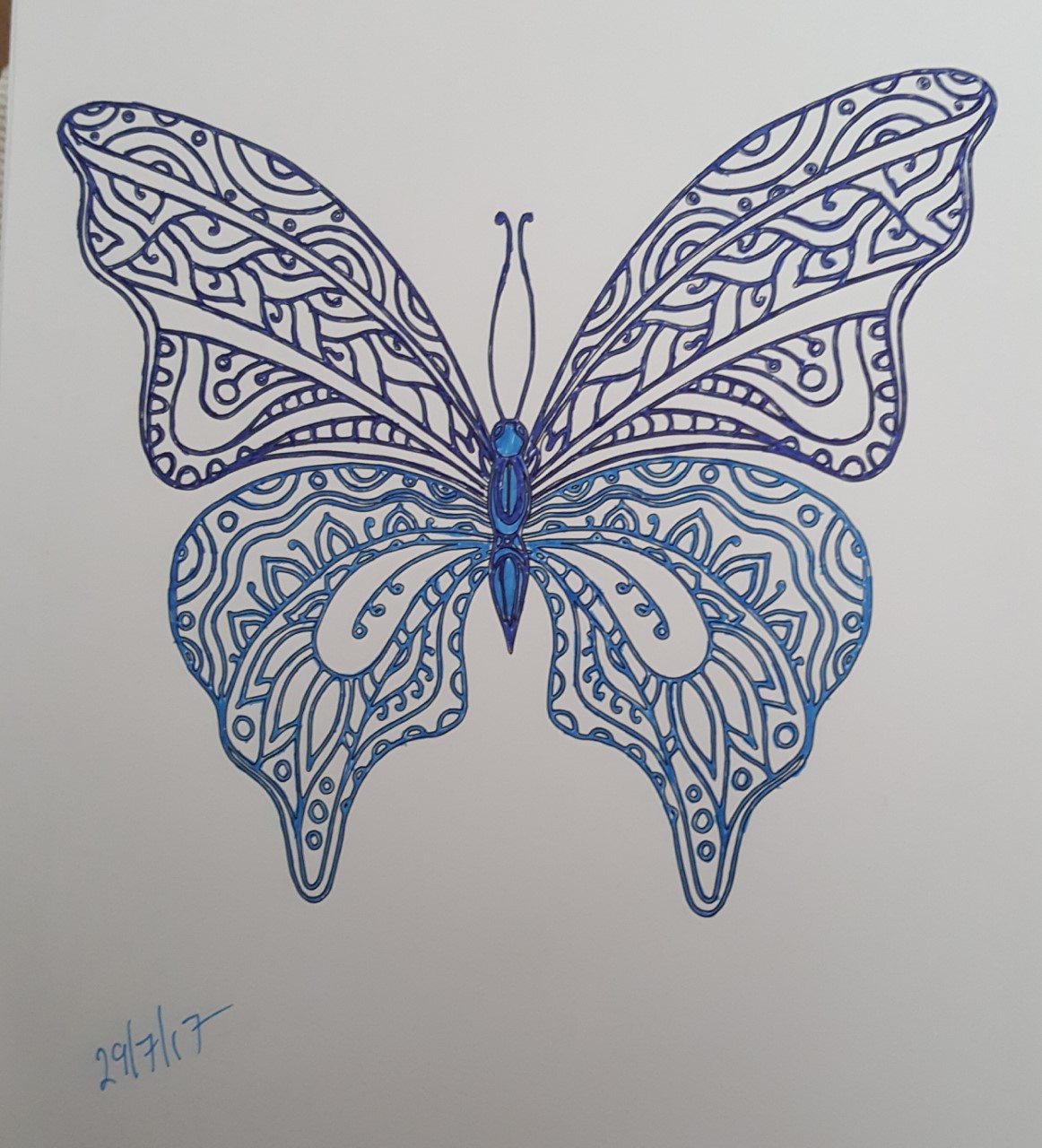This photograph captures a detailed illustration on a predominantly white surface, likely paper, which occupies about 97% of the image. In the top left corner, a small portion of a dark brown object is visible behind the paper. The illustration itself is a meticulously drawn butterfly. The top half of the butterfly's wings are rendered in a glossy dark blue ink, featuring an intricate pattern. This pattern is mirrored identically on both the left and right wings, suggesting we are viewing the butterfly from the back. The lower wings are depicted in a lighter blue hue, also mirror images of each other. The butterfly's body showcases a harmonious blend of dark and light blues. Notably, the butterfly has two long, elegant antennae extending upward. In the bottom left corner of the illustration, a date—handwritten in light blue ink—reads "29/7/17."